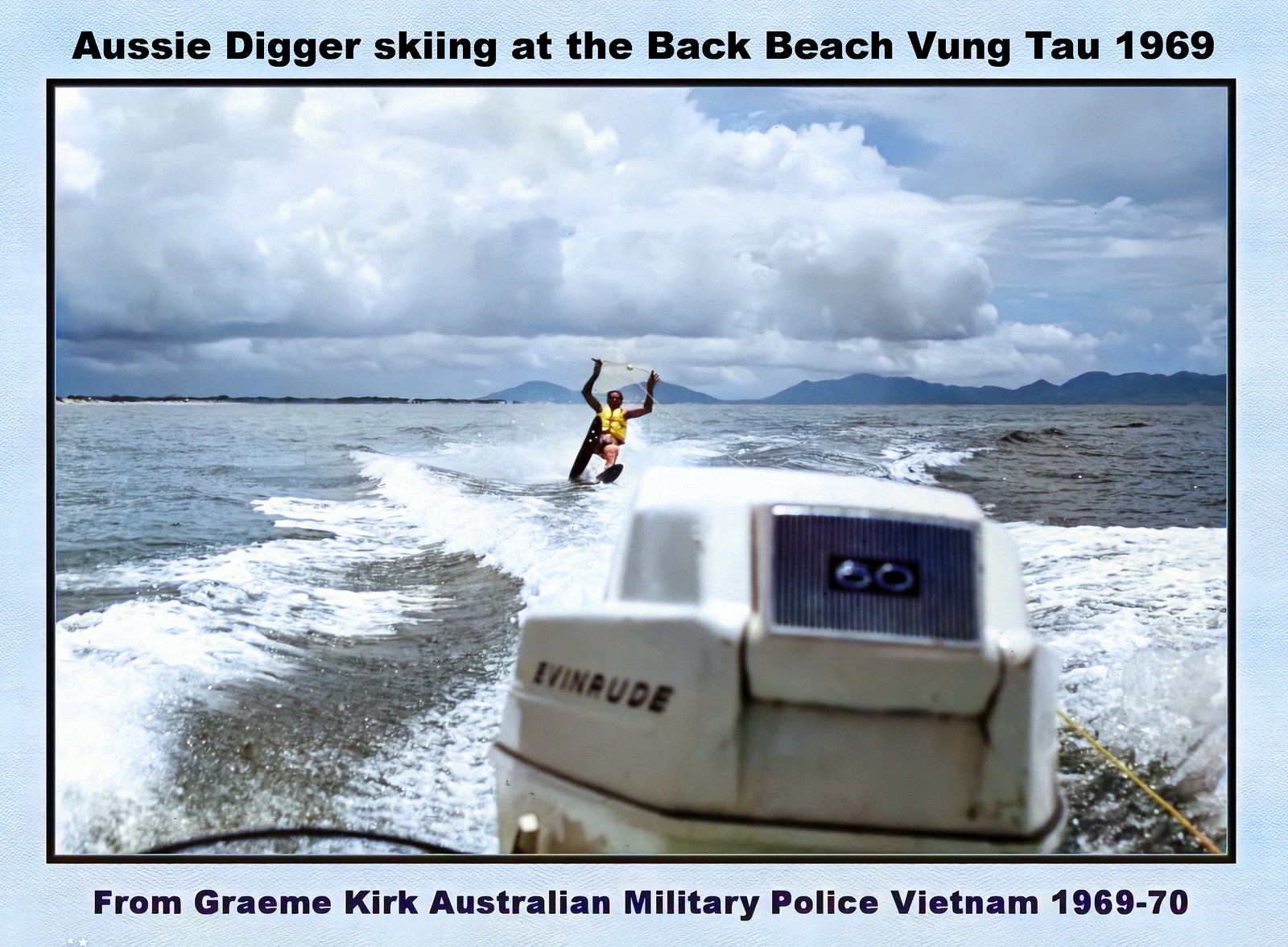This rectangular photograph, framed with a black border and matted with light blue, is headed by the text: "Aussie Digger Skiing" at Back Beach, Vung Tau, 1969. At the bottom, a caption reads: "Graham Kirk, Australian Military Police, Vietnam 1969-70." The image captures a dynamic scene taken from the vantage point of a boat, evidenced by the presence of an outboard motor in the foreground. In the distance, a water skier donning a yellow lifejacket is skillfully navigating through choppy waters, with one ski lifted into the air and the other gliding on the waves. The skier holds the tow rope high, maintaining balance amidst the substantial whitecaps, indicating turbulent and potentially frigid water, as suggested by its uninviting hue.